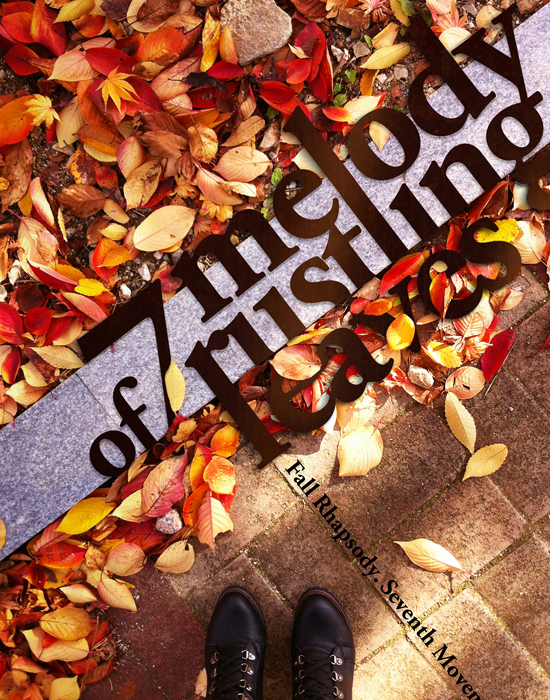The image showcases a vibrant autumn scene, predominantly featuring an array of colorful fall leaves in hues of yellow, orange, and red. These leaves scatter across the upper left section and part of the bottom left side of the image, laying on the ground. The scene is intersected by a diagonal paver path, which divides the vivid foliage. The path itself is gray, textured, and carved from stone. At the very bottom center of the image, a pair of black boots stands on a brown-pavered surface, giving the impression of someone standing there. Two textual elements overlay the image: in brown letters, "Seven Melody of Rustling Leaves" is displayed diagonally from the lower left to the upper right, and at the bottom, in black letters, going in the opposite diagonal direction, it reads "Fall Rhapsody, Seventh Movement." This juxtaposition of text and imagery suggests a flyer or visual motif celebrating the musicality and beauty of the autumn season.